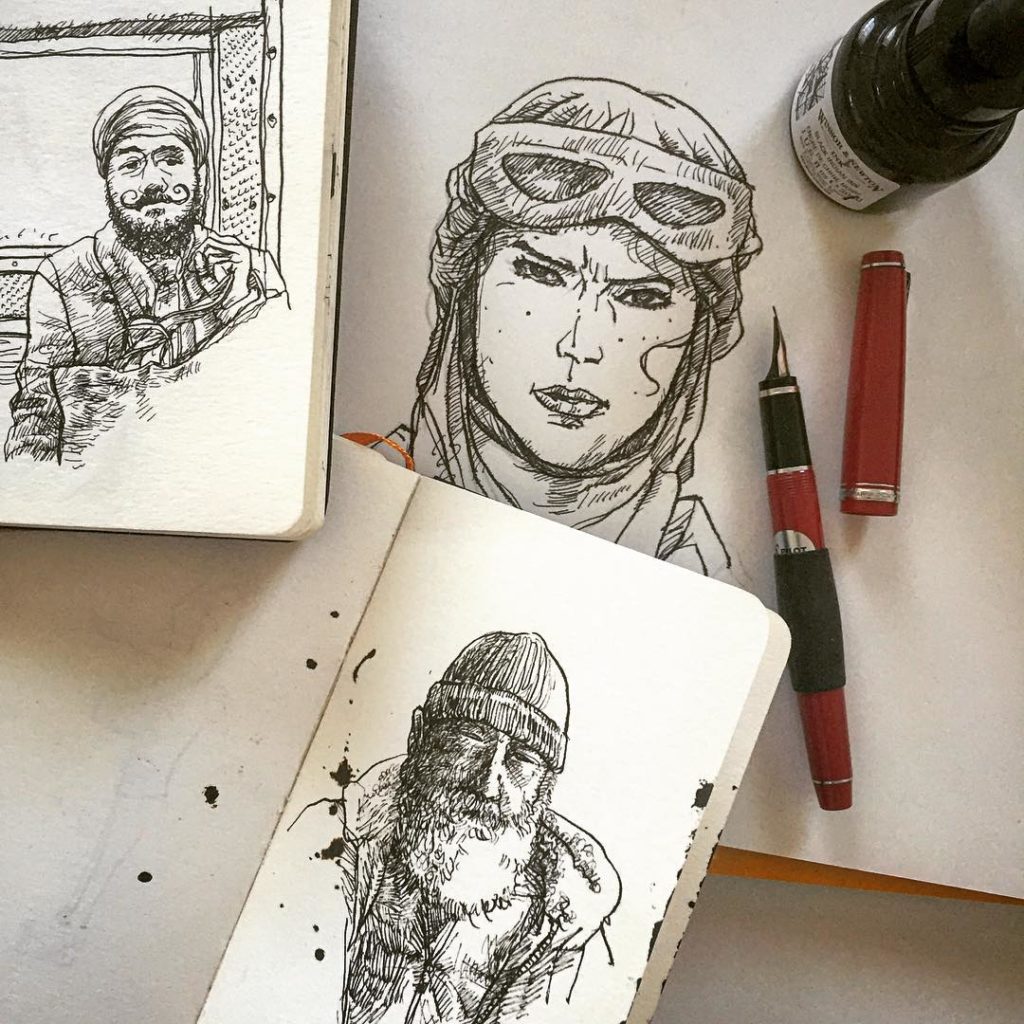This color photograph showcases an artist's workspace featuring three open journals stacked atop one another, with intricate black ink drawings made using an old-style reservoir ink pen. Each notebook is positioned to highlight a distinct illustration, framed by the accompanying tools of the trade: a long-pointed ink pen resting on the papers, and a large bottle of black ink stationed at the top right of the image.

The upper left corner displays a small journal depicting a detailed portrait of a man with a turban and a curly mustache, suggestive of Indian or Pakistani heritage. The middle journal contains a striking image of a stern-looking aviator, characterized by his balaclava and aviator goggles pushed up on his forehead, gazing intently. The bottom notebook features an elderly man with a long white beard, wearing a coat with a large collar and a toboggan, evoking the image of either a fisherman or perhaps a Viking. The artist has meticulously captured the essence and personality of each figure, from the expressive facial hair to the evocative attire, enhancing the depth and narrative of their characters.